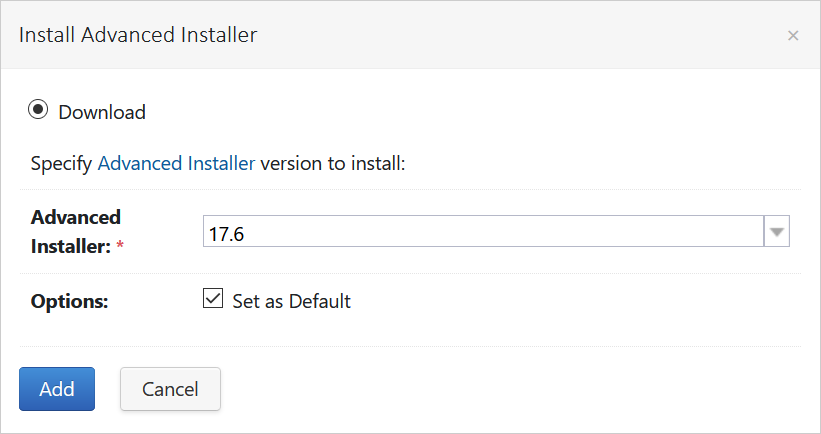In this image, we see a detailed screenshot featuring the installation interface for the Advanced Installer software. The screenshot itself is rectangular and horizontally elongated with a subtle light gray border. 

At the top, there's a light gray header bar with dark gray text in the upper left corner that reads "Install Advanced Installer."

Below this header, the primary background of the interface is a clean, solid white. On the left side, in dark gray text, the word "Download" is displayed, accompanied by a blackened circular icon to its left.

Further down, the text "Specify" appears, followed by "Advanced Installer" in blue text along with "version to install" in black text below it. The next line features "Advanced Installer" in bold black text, with a red asterisk immediately to the right, indicating a mandatory field.

To the right of this label, a form field is present, displaying the version number "17.6." This field includes a gray pull-down arrow to the far right, allowing for selection of different versions.

Below the form field, the word "Options" is written in bold black text on the left. To the right, there's a checkbox labeled "Set as default," which is checked off, indicating this option is selected.